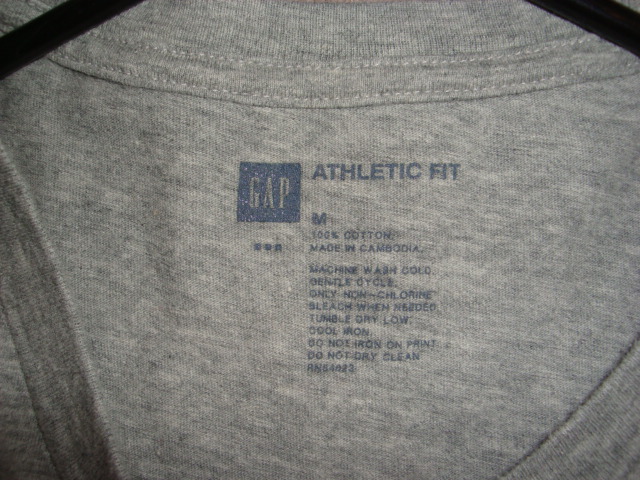In this image, we have a top-down view of the interior of a shirt, turned inside out. The garment, whose style cannot be confirmed as either a long-sleeve shirt or a t-shirt, features its branding printed directly onto the fabric rather than on a traditional tag. The prominent print is encased in a blue square, displaying the name "GAP" in bold white capital letters, indicating it’s from the GAP store. To the right of the GAP logo, the shirt is labeled as "Athletic Fit" in capital letters. Below this, the shirt size is denoted by a large letter "M" for medium. In smaller print, detailed care instructions are listed line by line: "100% cotton," "Made in Cambodia," "Machine wash cold," "Gentle cycle," "Only non-chlorine bleach when needed," "Tumble dry low," "Cool iron if needed," "Do not iron on print," and "Do not dry clean." The white stitching around the collar or neckline is clearly visible, emphasizing the inside-out aspect of the shirt.